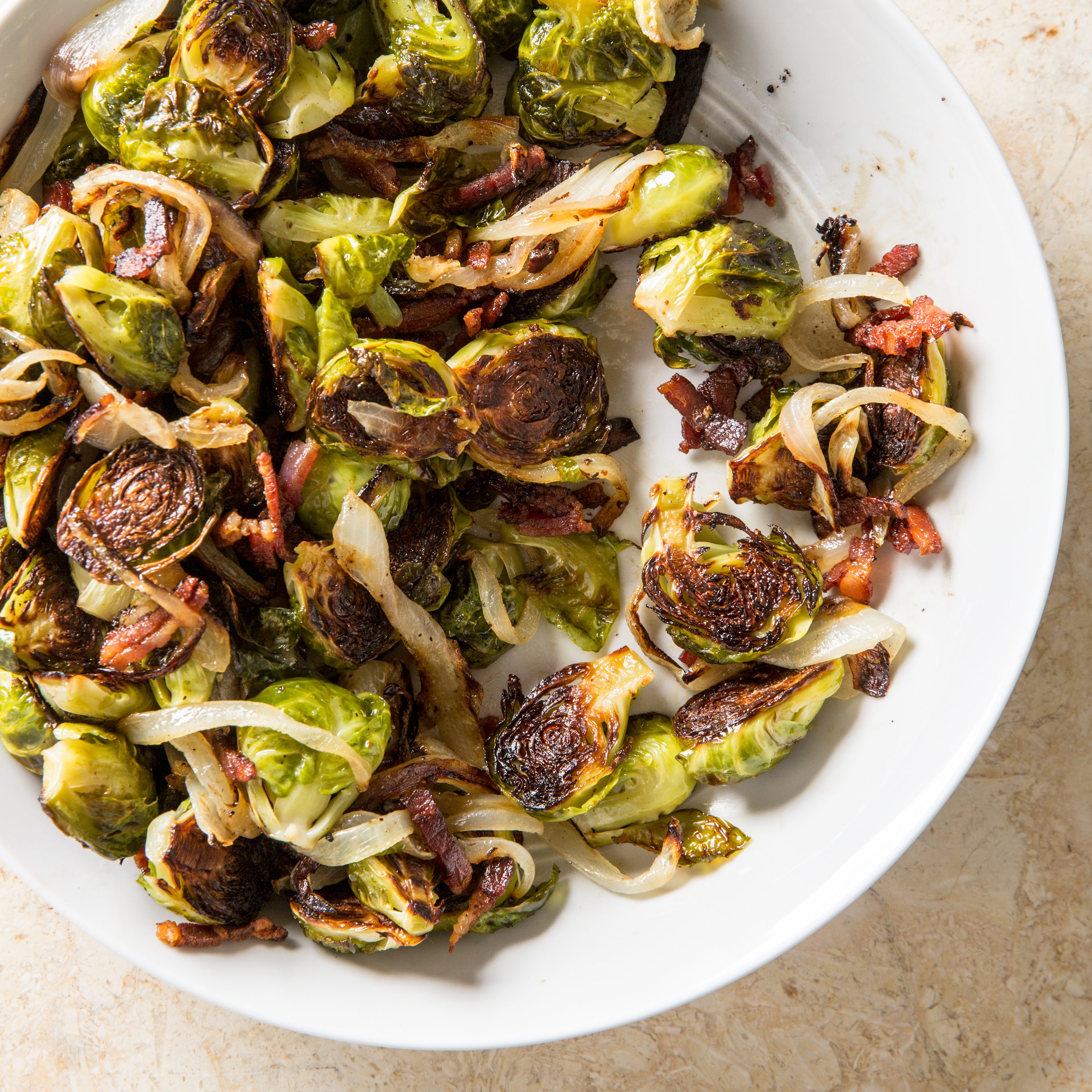A close-up image captures a meticulously arranged dish of roasted Brussels sprouts placed on a white, round bowl. The dish sits on a marble countertop. The Brussels sprouts are halved, displaying a rich range of colors from vibrant green to a dark, caramelized brown, indicating they were expertly roasted. Mixed among the Brussels sprouts are golden-brown, lightly cooked onions and crispy bits of bacon, adding complexity to the visual appeal. The white bowl, devoid of any color decorations, highlights the vibrant and appetizing colors of the food. The careful arrangement shows a concentration of Brussels sprouts to the left side of the bowl, while the upper right side features a sparser distribution, composing an artful balance that would be at home in a high-end recipe book.